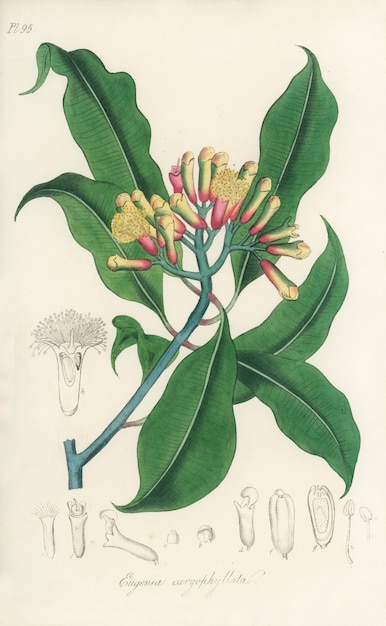The image is a detailed botanical illustration in portrait orientation, depicting a flowering plant or shrub. The central focus is a green stem from which six pointed, curly dark green leaves extend. Three leaves are positioned across the top, and three are below, with a few smaller leaves intertwined. The plant features a cluster of tubular-shaped flowers at the top, transitioning from dark pink at the base to cream-colored yellow at the tips. Only a few buds are partially opened while most remain closed. Surrounding the colored illustration, there are gray-scale sketches of various parts of the plant and seeds, contributing to the botanical style of the artwork. The background is a light ivory, enhancing the detailed and delicate nature of this vertical illustration.